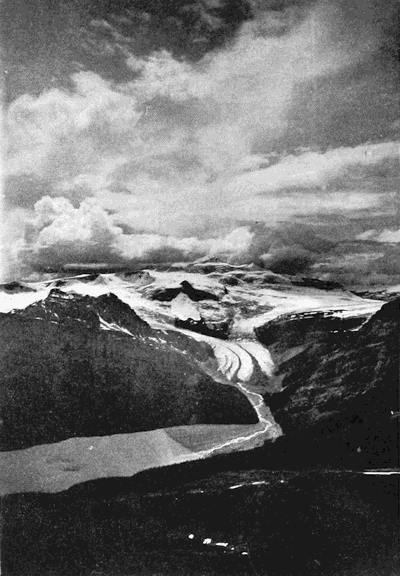This detailed description pertains to a seemingly old and grainy black and white aerial photograph or lithograph, featuring a panoramic view of a mountainous outdoor setting. The upper half of the image is dominated by a tumultuous sky with dark, stormy clouds mingling with billowy white clouds. The snow-capped, rocky mountains on either side blend almost seamlessly with these clouds, creating a stark contrast. A lighter grey feature, possibly a road or a river with a distinctive white path through its middle, winds through the rugged terrain below. In the foreground, the ground appears almost completely black, scattered with small white dots that might represent stones or flakes. The overall composition is devoid of vegetation, with the dark and light elements sharply contrasting in the grayscale spectrum, and there is a hint of a glacier nestled in the valley between the mountains.